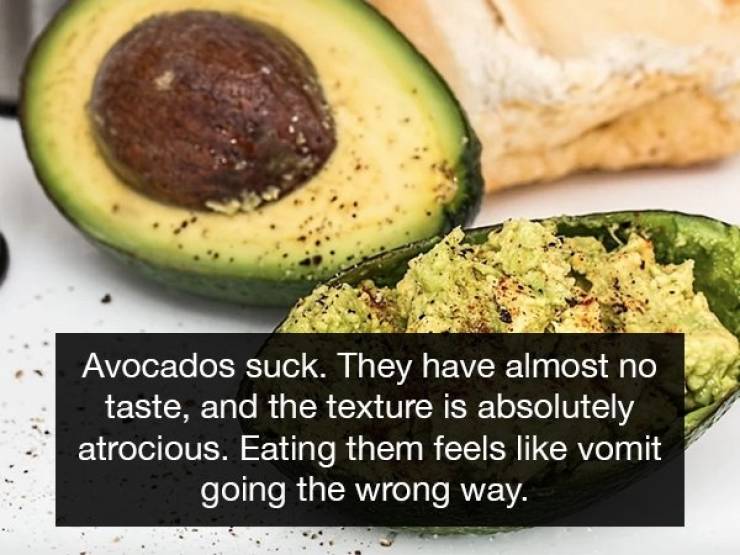This image features a meme with a bold, black rectangle at the bottom containing white, sans-serif text that reads, "Avocados suck. They have almost no taste, and the texture is absolutely atrocious. Eating them feels like vomit going the wrong way." The background showcases two avocado halves on a light gray or white surface. The upper left-hand corner displays the first half of the avocado, which prominently occupies the space extending towards the middle. This half contains a large brown seed at its center, surrounded by light green flesh sprinkled with black specks, likely pepper. The dark green peel of the avocado is visible along the edges. The other half of the avocado, taking up the middle to the lower right-hand corner, appears to be filled with a guacamole-like mixture, featuring both black and brown specks of spices, adding colorful seasoning throughout. The mixture is still housed within the avocado peel, and some seasonings are scattered on the surrounding surface. Additionally, in the top right-hand corner, there's an extra detail—a folded piece of bread with flour dusted over it.